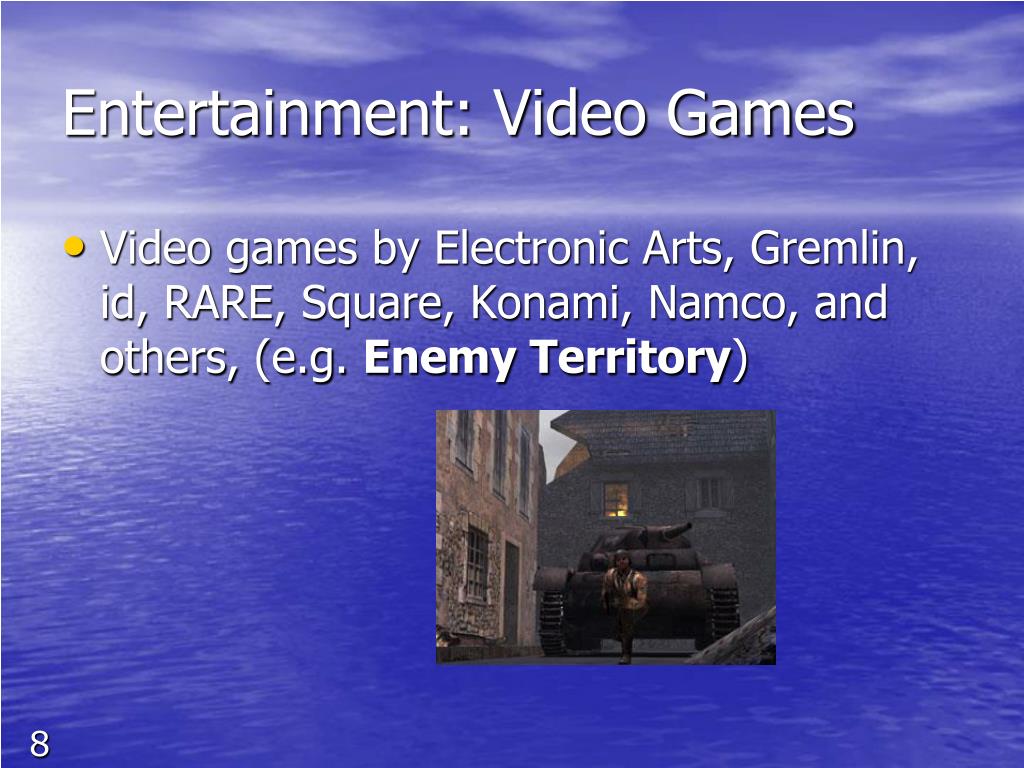The image features a vividly purple ocean and sky contrasting against wispy white clouds, lending a surreal, dreamlike quality to the scene. The ocean, with its purplish-blue hue, mirrors the sky above, while a subtle mist blurs the horizon. The text "Entertainment: Video Games" is prominently displayed at the top in white, followed by a bullet point list that reads "Video games by Electronic Arts, Gremlin, ID, Rare, Square, Konami, Namco, and others (e.g., Enemy Territory)." Positioned below this text is a small, detailed picture showcasing a rundown, tan-colored building on the left and a darker, blackish-brown building farther back. In front of these buildings stands a dark brown tank, beside which a soldier in black army gear, complete with a helmet and gun, is poised. The overall aesthetic suggests an early 2000s graphic design, synthetic and highly digital, reminiscent of classic PowerPoint slides. The slide combines a stark, digital background with informative text and a screenshot from the video game "Enemy Territory,” providing a compelling visual summary of video game entertainment.